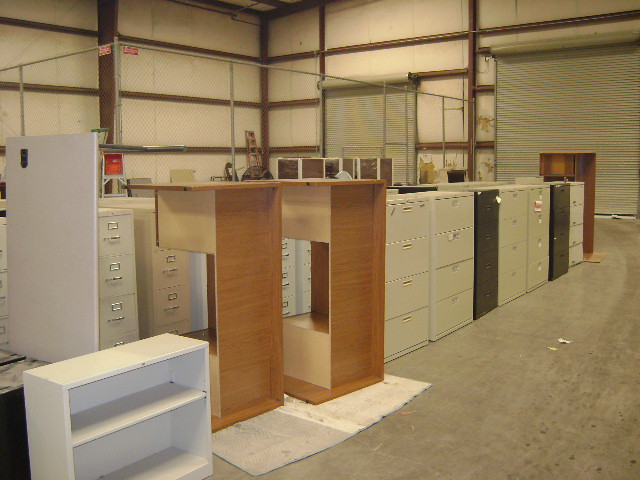Inside a spacious warehouse with large roller doors at the end, a collection of used office furniture is meticulously laid out on the bare concrete floor. Prominently featured are several four-drawer filing cabinets in varying colors, including black, white, and even tan, each with pull-out drawers. Alongside these cabinets are brown wooden desks, turned vertically on their sides, showcasing their plywood laminated tops. A white blanket supports one of these desks. Additionally, there are two-tier wooden bookshelves, resembling those commonly found in classrooms, standing upright. This warehouse scene is a detailed snapshot of an array of office furniture, all neatly organized and waiting for use.